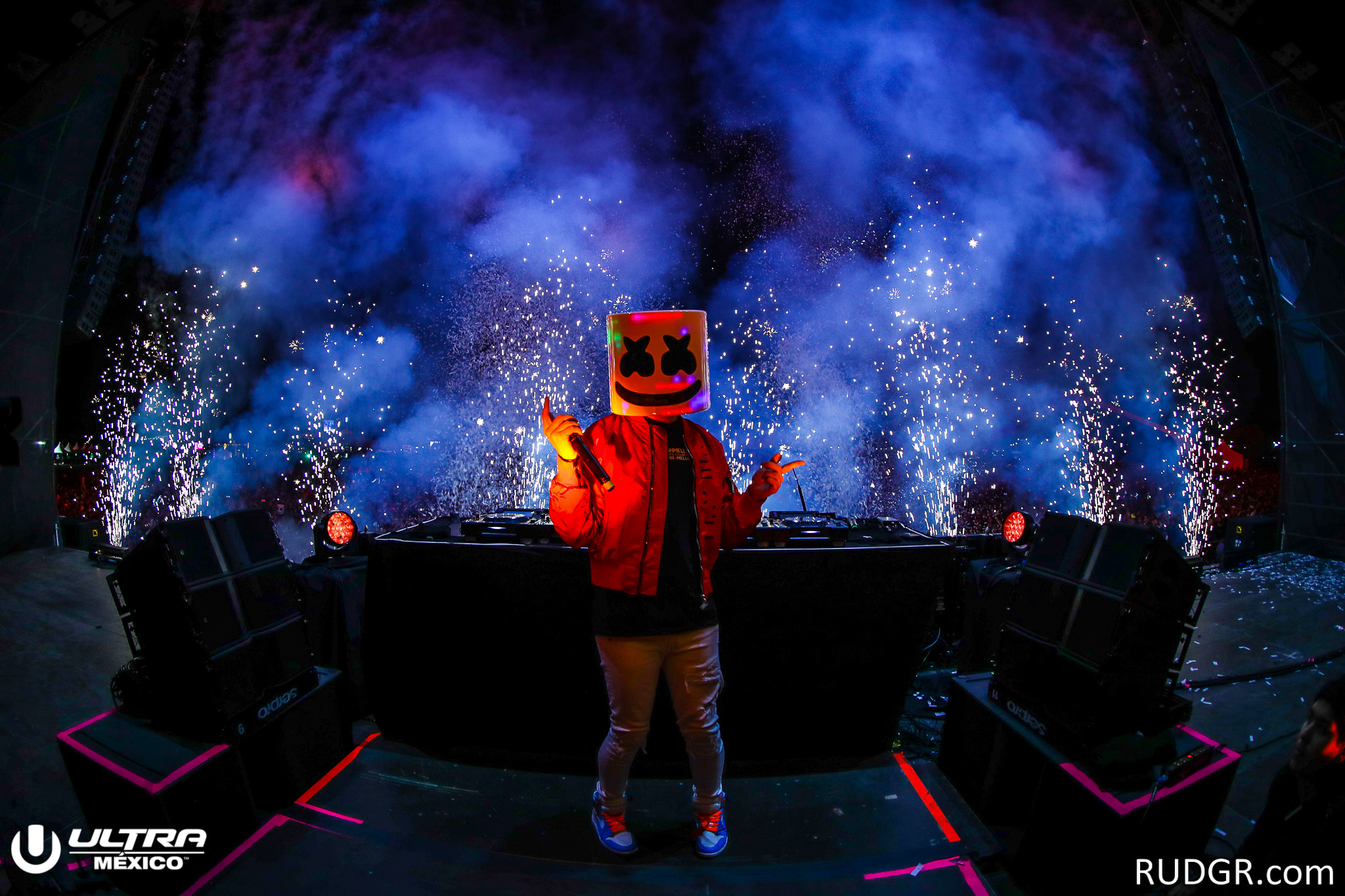A vibrant color photograph captures a dynamic DJ performance on stage. The focal point is a man, likely the DJ, dressed in a distinctive character outfit featuring a box with a smiley face drawn on it as his headpiece. He sports a red jacket over a black shirt, paired with khaki pants and eye-catching blue and white sneakers adorned with orange laces. Surrounding him is an array of audio equipment, including DJ turntables, speakers, and other electronic gear. The stage is accented with striking red and purple neon tape, enhancing the visual appeal. In the background, a spectacular pyrotechnics display is in full swing, emitting bright lights and creating a thick cloud of blue smoke, adding to the electrifying atmosphere of the performance.